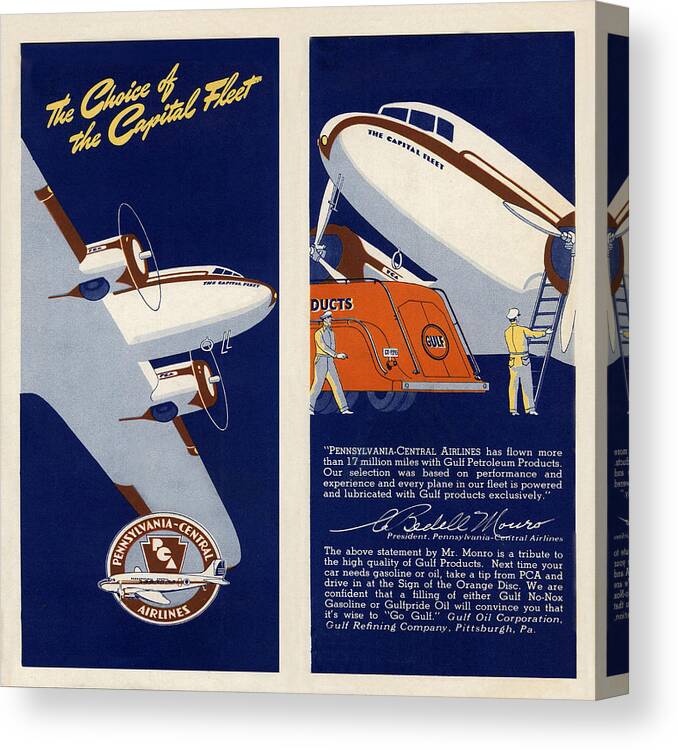The image showcases a box set against a white background, featuring two rectangular panels in navy blue that display illustrations of a white airplane with brown trimmings. The airplane, a white propeller-driven model with "Pennsylvania Central Airlines" and "The Capital Fleet" branding, is prominently featured.

On the left panel, cursive yellow text at the top says, "The choice of the Capital Fleet." Below the text, a white propeller airplane is depicted flying in the sky, with a central logo that reads "Pennsylvania Central Airlines."

The right panel shows the same airplane landed, with the propellers stationary. People are servicing the airplane: one person is positioned on a ladder against the engine, and another person is walking towards it. There is also an orange machine next to the airplane. In this panel, white text reads: "Pennsylvania Central Airlines has flown more than 17 million miles with Gulf Petroleum products. Our selection was based on performance and experience, and every plane in our fleet is powered and lubricated with Gulf products exclusively. The statement by Mr. Monroe is a tribute to the high quality of Gulf products. Next time your car needs gasoline or oil, take a trip from PCA and drive in the sign of the orange disc. We are confident that a filling of either Gulf, NONOX gasoline, or Gulf Pride oil will convince you that it's wise to go Gulf. Gulf Oil Corporation, Gulf Refining Company, Pittsburgh, PA."